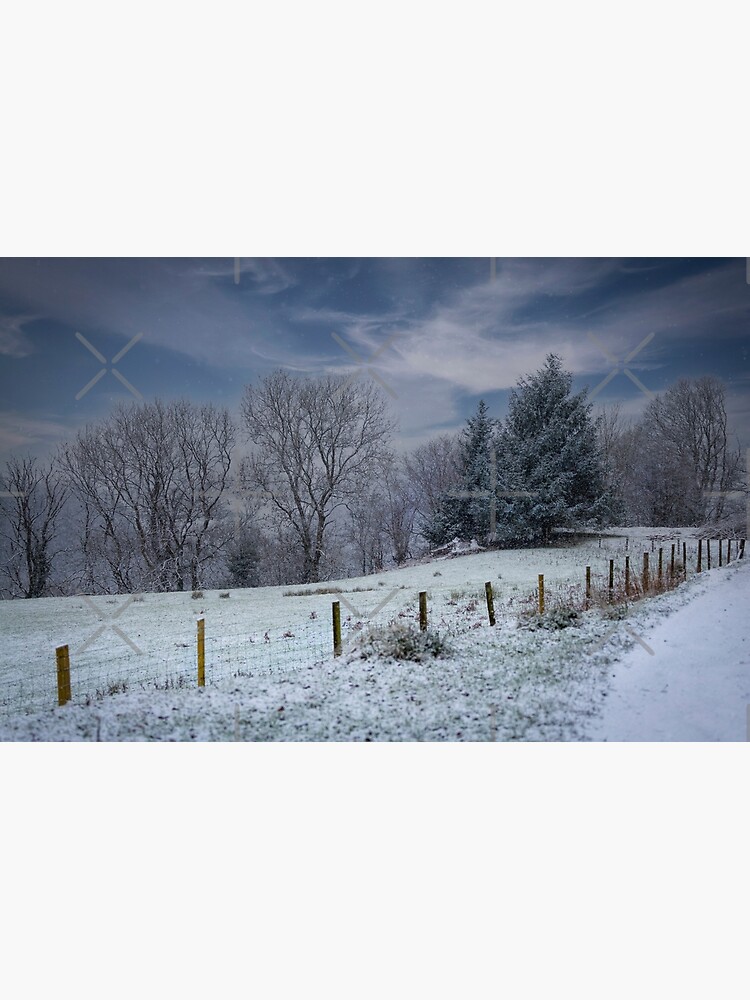This detailed photograph captures a picturesque winter scene in a snowy area featuring a mix of bare hardwood trees and beautiful evergreen trees sprinkled with snow. The evergreens, resembling Christmas trees, stand out vividly against the predominantly white landscape. In the background, trees without leaves extend into the distance, framing the scene and reinforcing the wintry feel. The ground is blanketed in snow, though small patches of green grass poke through, particularly on a slight hill in the foreground. A wooden fence with wire mesh runs into the distance from the center towards the right side of the image, where it borders a snow-covered road that is partially visible. The sky above is a blend of blue with wispy white clouds, creating a serene backdrop. Interestingly, several faint gray Xs are superimposed across the photograph, suggesting it might be a marked sample or print. Overall, this view captures the quiet beauty of a winter's day.